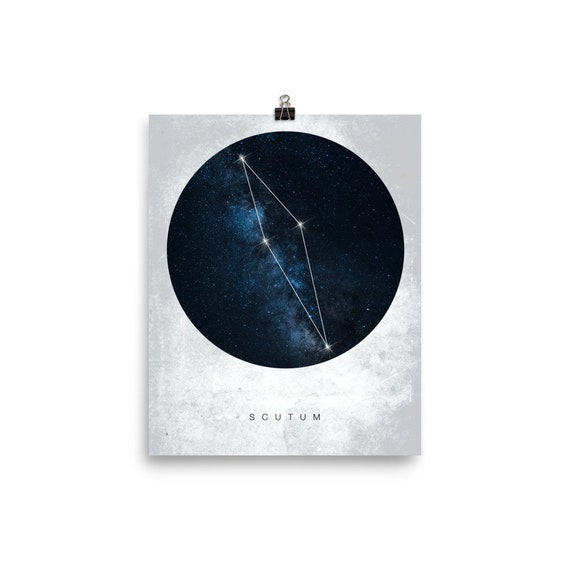The image depicts a small photograph of what appears to be the cover of a book. The book cover features a predominantly white background, which includes shades of gray. Near the bottom of the cover, the word "SCUTUM" is written in thin black, capital letters. The central focus of the cover is a dark blue circle illustrating a starry night sky, populated with numerous stars. Particularly highlighted are four very bright white stars, arranged in a long diamond shape and connected by white lines, indicating a constellation. At the top of the book cover, a black binder clip with metal prongs is attached, seemingly used to hang or hold the book in place on a wall.